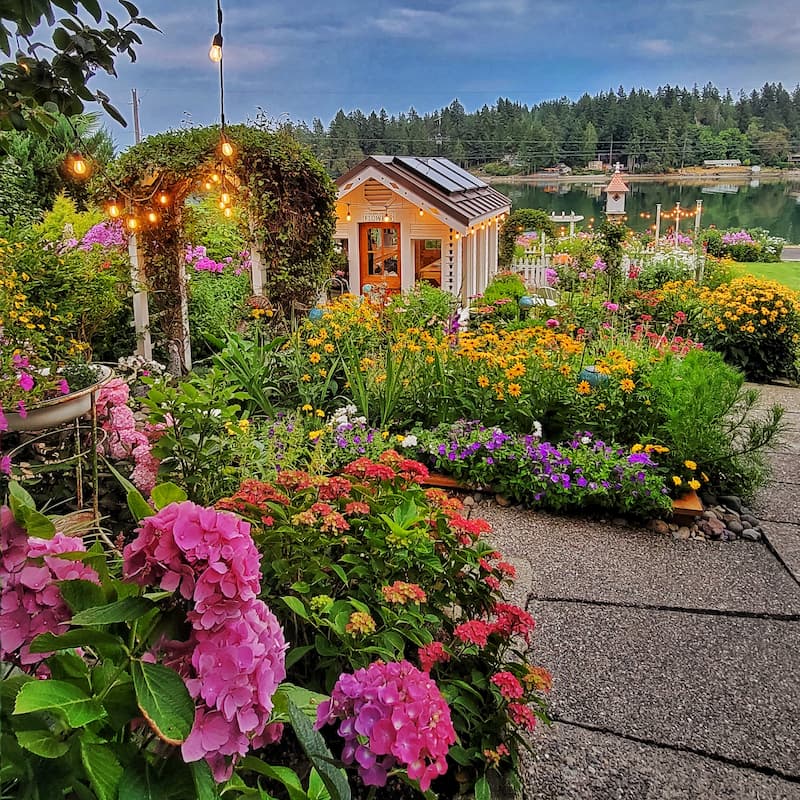The vibrant image showcases a bustling garden store set center stage, housed in a small, wooden structure with a brown door and solar panels adorning its roof. Surrounding the store, a lush array of flowers in full bloom adds a riot of color. In the lower left corner, a medley of purple and light purple flowers protrudes from verdant green leaves. Accompanying them are clusters of red and pink flowers and a charming flower pot on a stand, sprouting yellow and purple blossoms. A trellis to the left burgeons with climbing flowers, festooned with lights that weave around its structure.

In front of the store, on a darker, speckled concrete walkway, an explosion of floral diversity continues. Purple, yellow, and pink blooms — including hydrangeas, verbena, and peonies — interlace with petunias and yellow coneflowers, creating a dazzling tapestry of colors. The garden stretches outward to a tranquil pond or lake in the background, which is mirror-flat and bordered by distant dwellings and a dense forest.

Further enhancing the scenic beauty, additional lights are strung near a classic white picket fence and a light brown steeple atop a white building rises in the far distance, adding a quaint charm to the setting. The entire scene is serene and picturesque, brimming with nature's splendor and an air of peaceful seclusion, possibly suggesting a lakeside retreat.